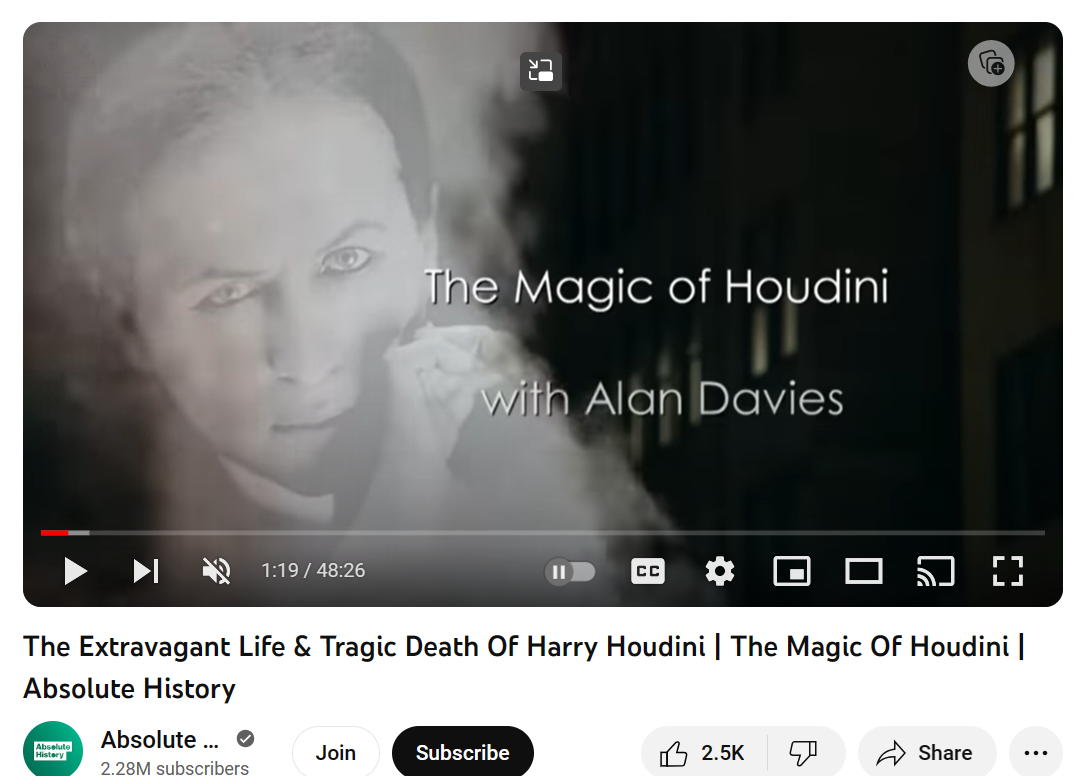The image is a paused screenshot from a YouTube video titled "The Extravagant Life and Tragic Death of Harry Houdini, The Magic of Houdini" from the Absolute History channel, which has 2.28 million subscribers. The video, currently paused at 1 minute and 19 seconds out of a total duration of 48 minutes and 26 seconds, features a black-and-white photo of a white man, presumably Harry Houdini, with a scowling expression and one eyebrow arched, standing in a shadowy, fog-filled setting that resembles a warehouse. In the middle, slightly to the right, white text reads "The Magic of Houdini with Alan Davies." Below the video player, there are standard YouTube controls and icons, including the join button, subscribe button, thumbs up (2.5K likes), thumbs down, share button, and additional menu options. The Absolute History logo is also visible.